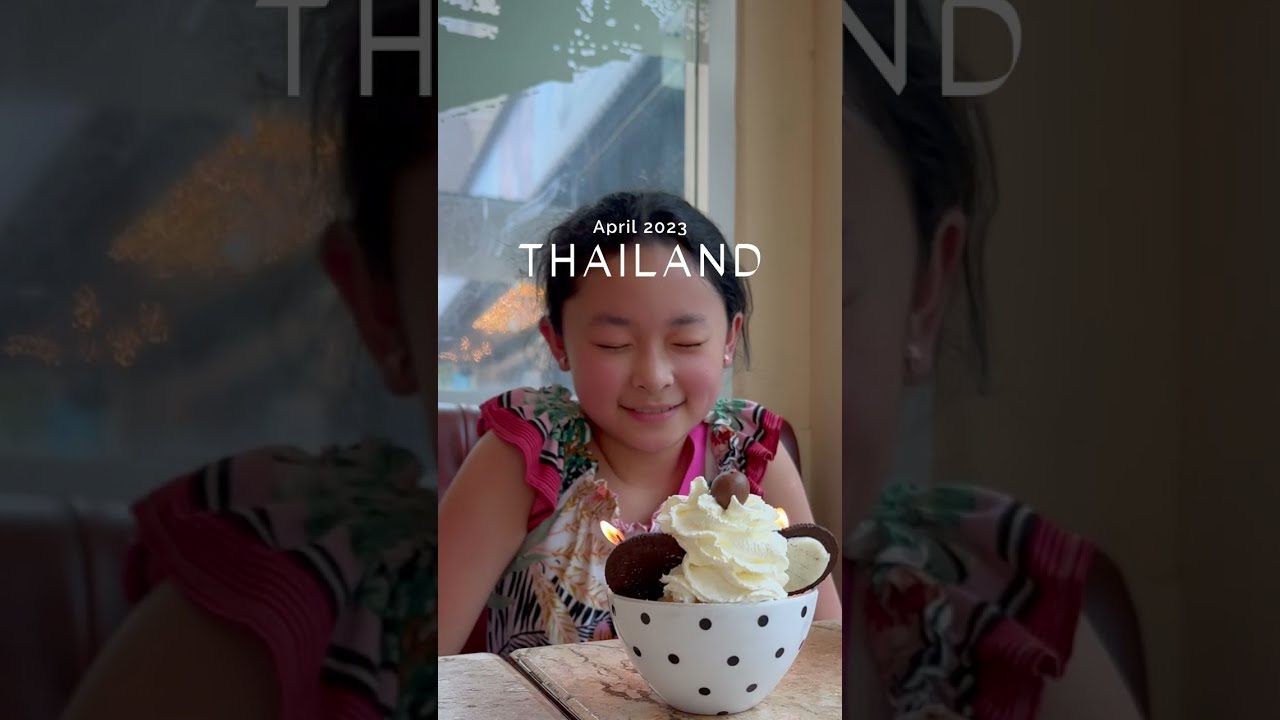In the center of the photograph, there's a smaller, clearer image that says "April 2023, Thailand." It features a young Asian girl with her eyes closed and a smile on her face. She has black hair pulled back and is wearing earrings. Her dress is a burst of colors with shades of pink, green, white, black, and frilly sleeves accented with pink trim. She sits at a table with a large white bowl with black polka dots in front of her. The bowl is piled high with whipped cream, chocolate cookies, and a piece of chocolate, possibly suggesting an ice cream dessert. A small lit candle, hinting at a celebration such as a birthday, is also in the bowl. 

The central photo is vividly bright and sharp, contrasting with the diffused images on either side. These side images are blurred and look like they're seen through a darkened glass, mirroring parts of the girl's body but omitting the elaborate dessert centerpiece. The background images emphasize the prominence and clarity of the central photograph, creating a layered composition that draws focus to the detailed and joyful expression of the young girl enjoying her treat.